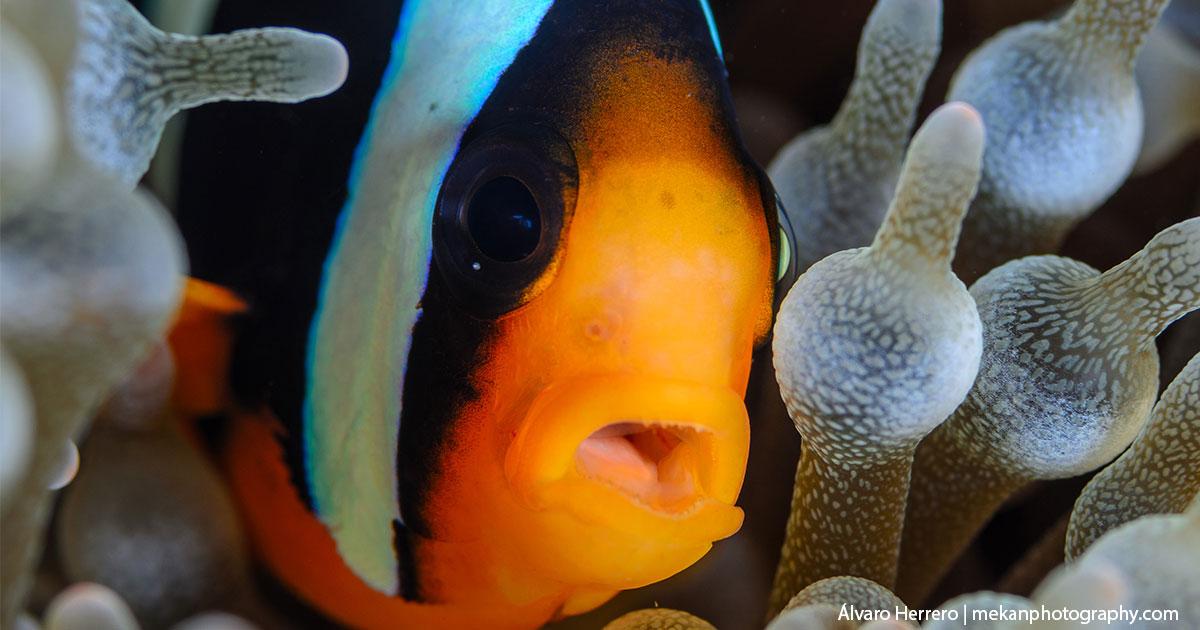This close-up image, taken underwater, showcases a vividly detailed small fish, identified potentially as a clownfish, set against an illuminated underwater backdrop. The picture, attributed to Alvaro Herrero MackinPhotography.com, captures the fish with its mouth open, emphasizing its black pupils and prominent eyes. The fish's body is oval and flounder-like, with thin, almost translucent scales. The predominant color is black, with a distinct bright turquoise stripe running across its head and some additional black markings. Its underbelly, mouth, and areas around the face are adorned with a yellowish-orange hue. Its scales display a gradient from orange around the mouth and belly to black across the top and sides of its face. The fish has a large white stripe positioned between the orange and black sections, enhancing the impression that it might be a clownfish. It is surrounded by bulbous, tube-like sea plants or barnacles, which appear semi-transparent, bluish, and dotted with dark brown spots. These sea plants look almost self-illuminated, with a unique bulb and nipple-like structure at the top, adding to the enchanting underwater scene.